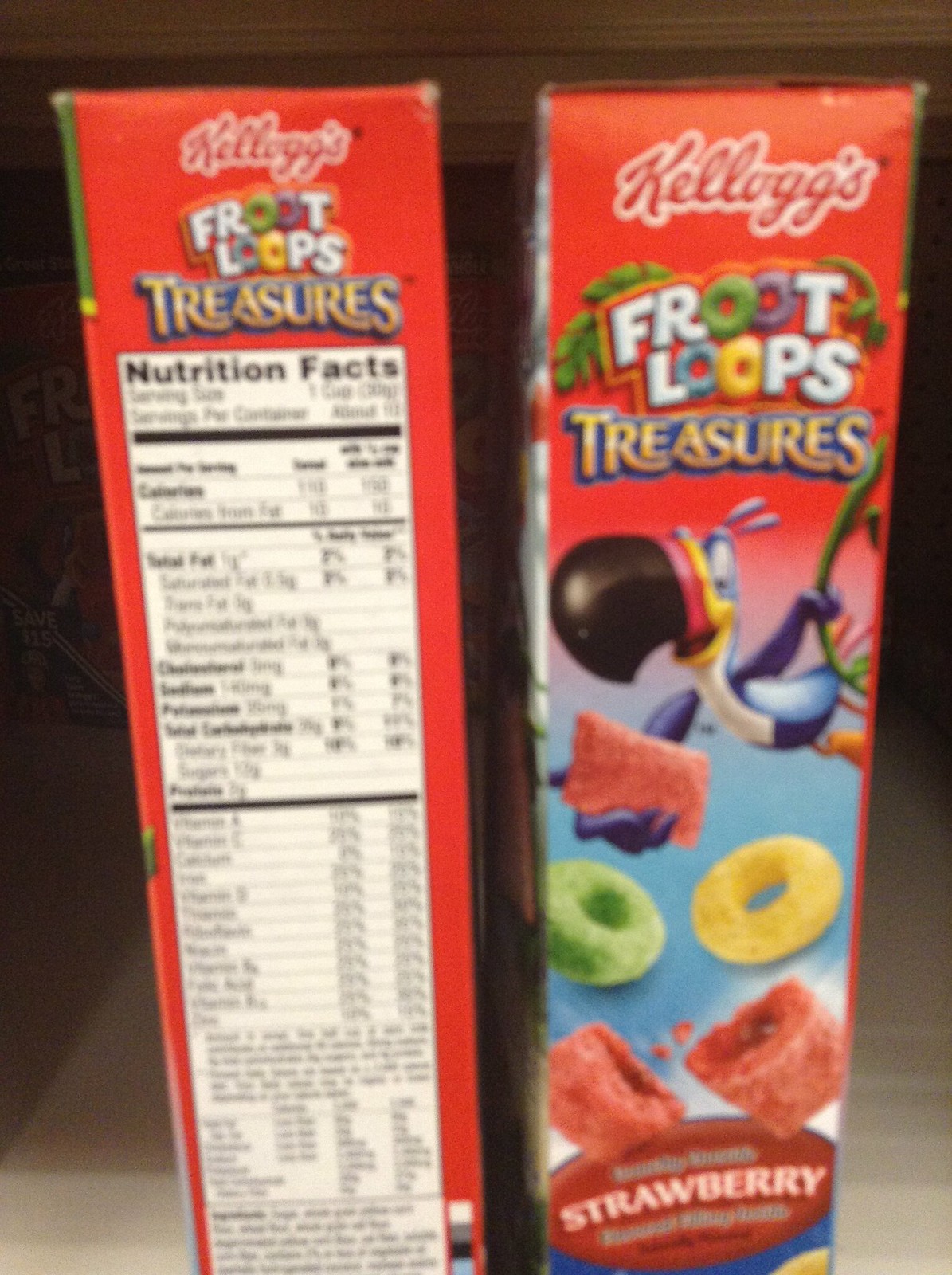This image features two boxes of Kellogg's Froot Loops Treasures. The boxes are predominantly red. The left side of the image showcases a side of one box filled with nutrition facts information, though the text is blurry and difficult to read. The nutrition facts section occupies the entire side of the box. 

At the top of the front and side panels, the brand name "Kellogg's Treasures" is displayed in vibrant, multicolored text. The right side of the image highlights the front of the second box, which is more visually engaging. It depicts the lively character Toucan Sam, either flying or swinging from a vine, having just scooped up a red cereal piece.

The front view also showcases a variety of colorful, treasure-shaped cereal pieces in green, yellow, and red. Notably, there is a red strawberry-flavored cereal piece that is broken in half, revealing a detailed view of its inside texture. The design of the box creatively emphasizes the fun and playful nature of the cereal while spotlighting the product's colorful and appealing pieces.